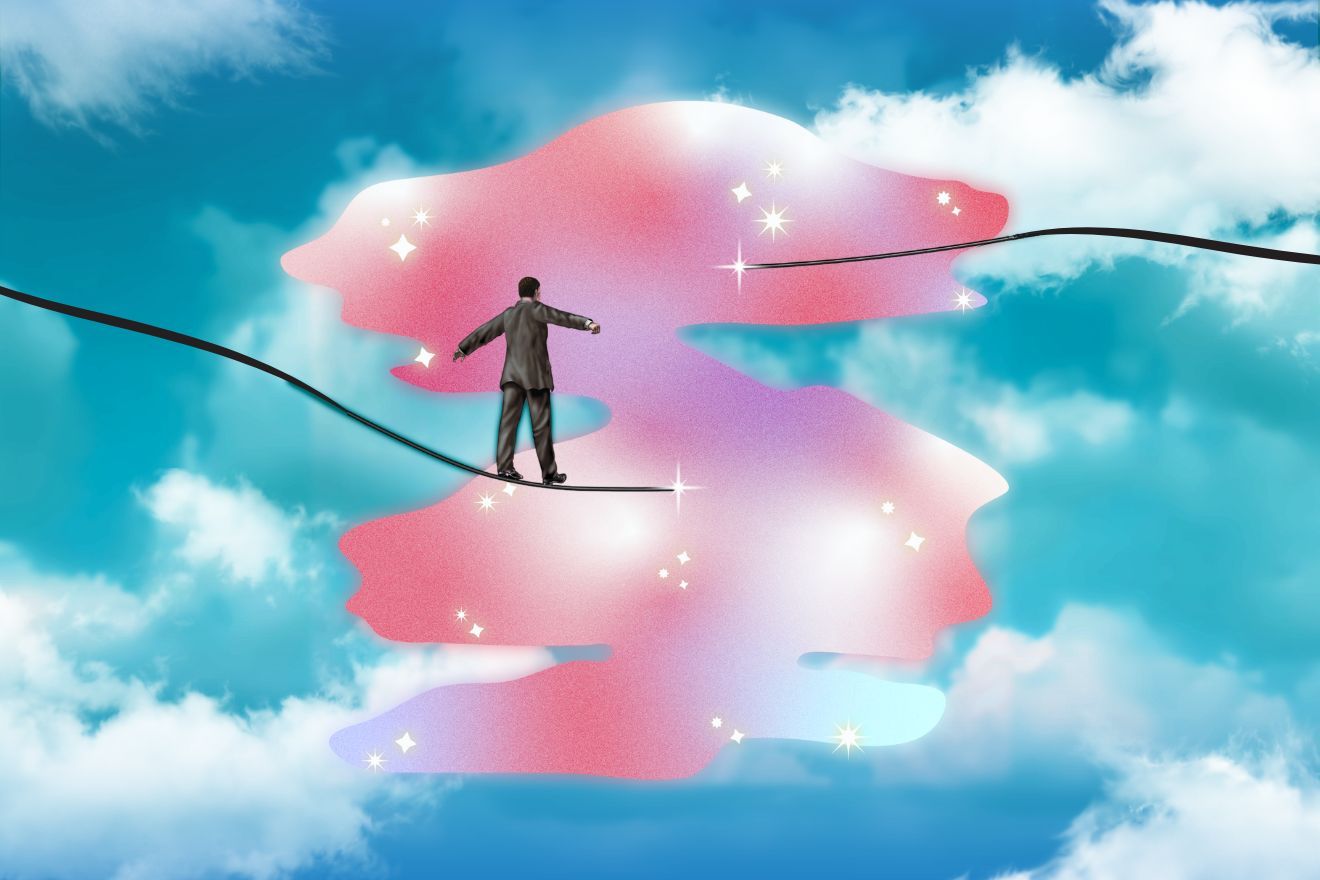The image is an artistic depiction set against a serene blue sky filled with scattered white clouds congregating at the upper left and right, and also at the bottom. Central to the composition is a man, dressed in a full gray suit, walking across a black line that resembles a tightrope. His arms are outstretched for balance as if traversing an actual tightrope high in the sky. The scene is further dramatized by an ink-like pink spill adorned with sparkling, diamond-shaped stars that are white and gold, positioned prominently in the middle of the image. The overall style appears to be digital artwork, perhaps watercolor or oil-based, evoking a sense of floating through a dreamscape.